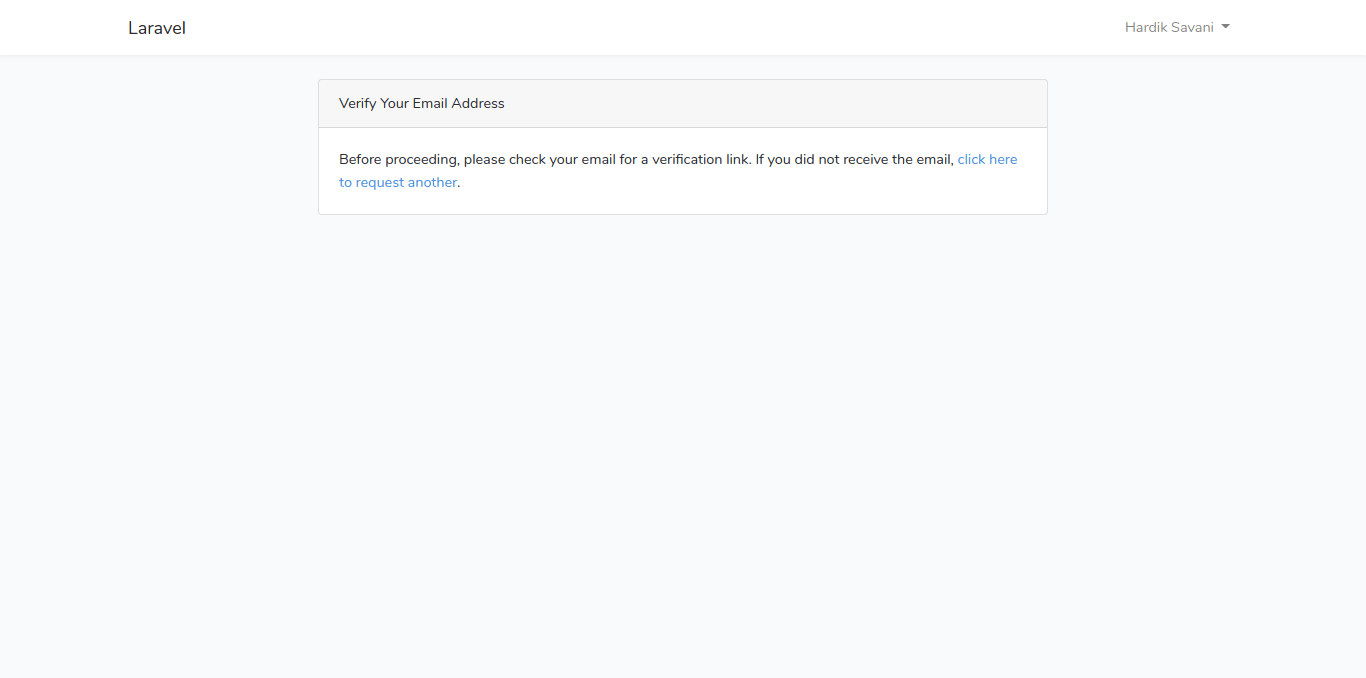The image depicts a webpage with a minimalist design primarily using shades of gray and white. Across the top, there is a white horizontal stripe running from the upper left to the upper right corner. On the left side of this stripe, the word "LARAVEL" is prominently displayed in uppercase letters. On the right side, a user profile name, "HARDIKSAVANI," is visible alongside a dropdown arrow, which likely offers additional options such as logging off.

Below this white header, the rest of the page features a very light gray background. Centrally positioned on the upper part of the page are two distinct rows. The first row is slightly darker gray and contains bold black text stating, "Verify Your Email Address." Directly below this, in the second row, the message "Before proceeding, please check your email for a verification link. If you did not receive the email, click here to request another," is written in bold black text on a white background. The phrase "click here to request another" is highlighted in blue, indicating it is a clickable link to resend the verification email.

The two rows containing the verification message are encased in a very light gray border and are separated by a light gray horizontal line, maintaining a clean and organized layout.